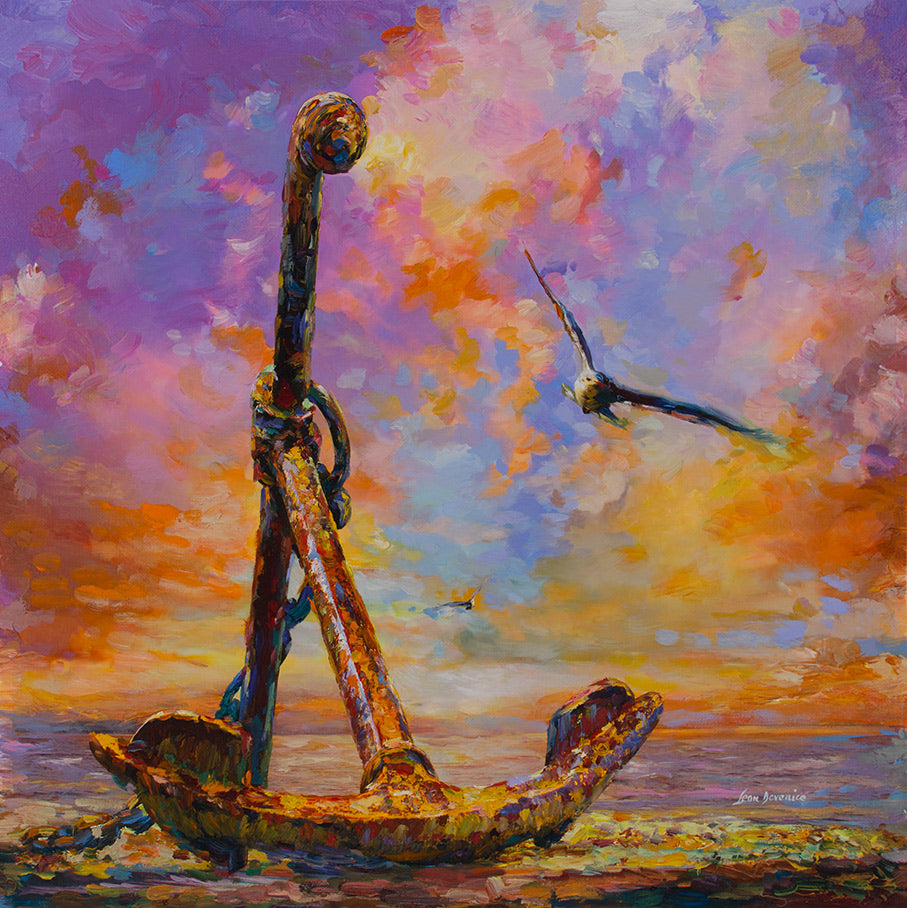This detailed and vibrant Impressionist oil painting captures a rusty anchor prominently positioned on the shore, tied to a metal pole with a chain. The anchor, in shades of brown, orange, yellow, and black, exhibits a worn, reflective surface, evoking a sense of age and history. In the sky above, two large birds, one resembling an owl and the other a seagull, soar against a backdrop of a vividly colorful sunset. The sky, painted with patches of orange, red, yellow, light blue, and purple, reflects over a vast body of water, suggesting a serene evening by the sea. The artist's signature, which appears to read something like "iron Devonese," is inscribed in white in the bottom right corner.